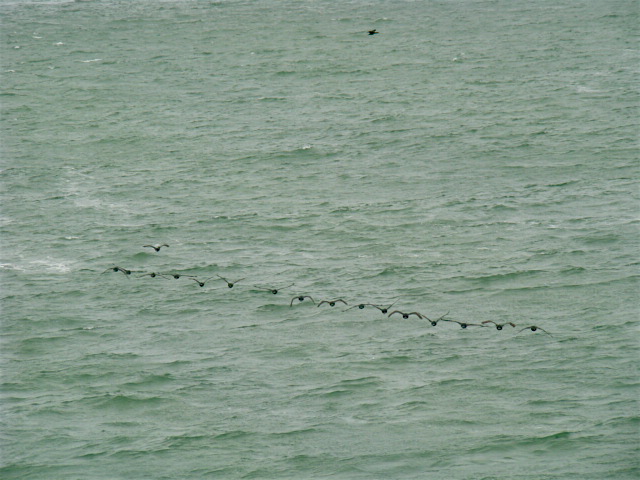This is a square color photograph of a grayish-green, slightly rough sea with subtle white caps. The absence of sky and any text places all focus on the water and the birds. Approximately 15 small black seabirds are flying in a straight horizontal formation about halfway down the frame, all with wings open, facing the viewer. One solitary bird flies just above this tight formation, appearing as if it's lagging behind. Near the top left of the frame, another bird is separate from the main group. Additionally, at the very top of the image, about half an inch from the edge, there is a black object in the water, possibly another bird. The dull, greenish hue of the ocean suggests an overcast day with no direct sunlight.